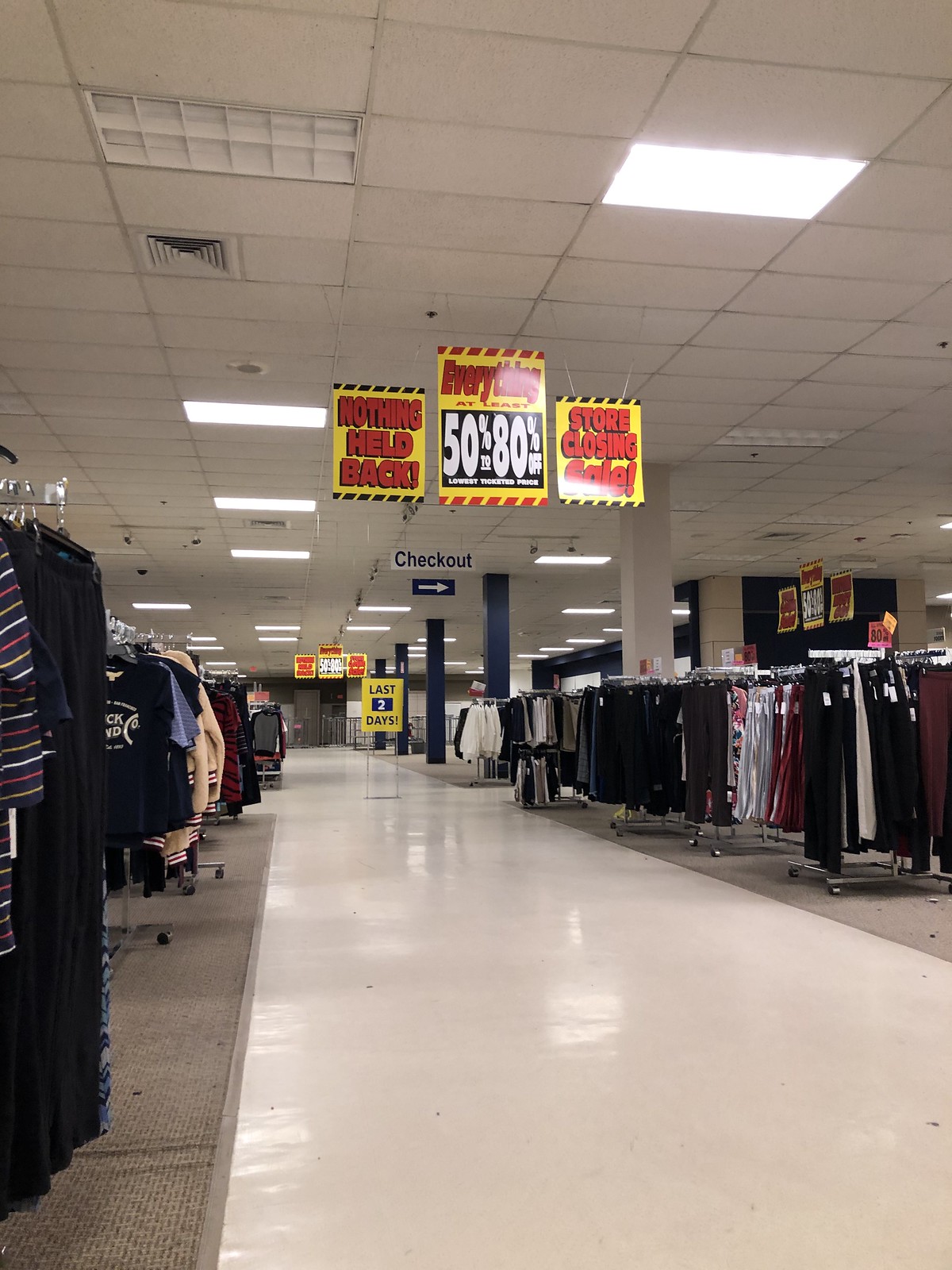This rectangular portrait photograph captures a department store undergoing a significant sale event. At the ceiling level, three prominent signs are aligned horizontally. The sign on the left, with a yellow background and bold red font, declares "Nothing Held Back." The central sign features the word "Everything" in striking red letters, complemented by a bold statement of "50% to 80% Off" in white font against a stark black background. The rightmost sign, mirroring the left sign's color scheme, announces a "Store Closing Sale" in red font on a yellow backdrop.

The photograph is taken from a straight-ahead angle, providing a comprehensive view from the floor to the ceiling. The layout includes clothing racks lining both sides of the image, filled with various garments. The store's floor is a combination of white tiles and light gray carpeting in the areas where the clothing racks stand. This detailed setup emphasizes the urgency and magnitude of the sales event happening in the store.